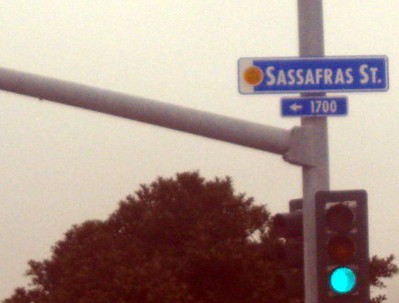The image captures a nostalgic scene, reminiscent of the 1980s, at a busy intersection under a completely overcast, grayish sky with no hint of blue. Dominating the right-hand side of the frame, there are two traffic lights mounted on a silver pole. The traffic light facing the viewer is illuminated with a bright green light at the bottom position, indicating it's safe to go. The second traffic light, which points towards the opposite side of the intersection, is not visible from this angle but is presumably red.

A second silver pole extends diagonally upwards to the left from the main pole and supports two blue street signs with white text. The upper sign reads "Sassafras Street," accompanied by a small circular icon. Below it, the second sign features a right-pointing arrow and the number "1700." Adding a touch of nature to the scene, the bottom of the image reveals the top of a green tree.

This detailed capture highlights the interplay between urban infrastructure and natural elements under a dreary, cloud-filled sky, evoking a sense of old-time urban tranquility.